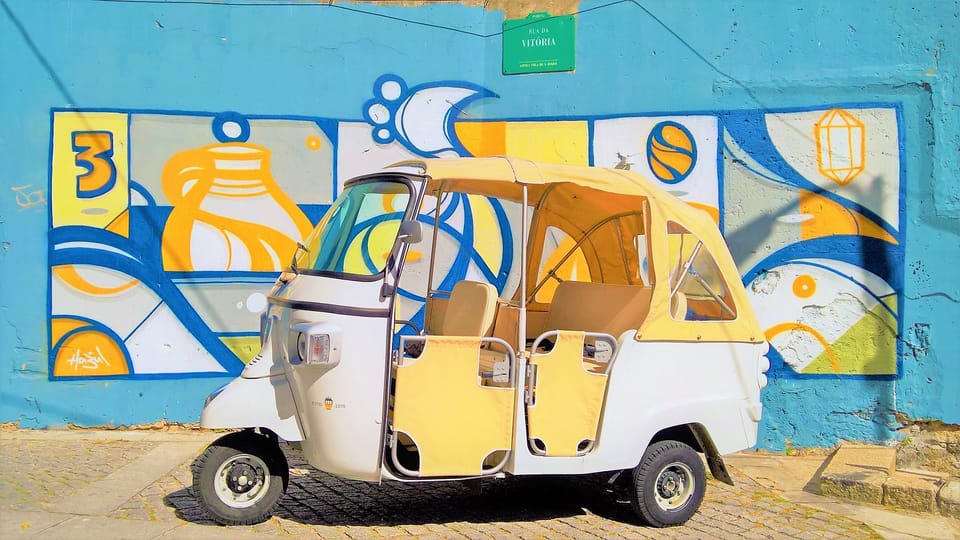In front of an aquamarine blue wall adorned with a vibrant mural featuring the number "3," abstract shapes like a lamp, a diamond, an orange water bottle, and swirling patterns in yellow, blue, gray, and white, sits a uniquely whimsical electric cart that almost resembles a small taxi or golf cart. The mural creates a lively backdrop with its colorful mosaic of elements, including what appears to be a volleyball and jug.

The cart, gleaming in its shiny white paint, sports a curvy front with a large arched window for the driver. A distinctive nose-like protuberance and headlights give the cart a charmingly anthropomorphic face. Its tiny front wheel is encased in a black tire with a white hub, mirroring the larger wheels at the back.

Made for leisurely rides, the vehicle features two passenger seats at the back, encased in light yellow plastic with matching canvas coverings. The framework consists of metal tube doors draped with yellow fabric, offering a convertible-like experience. A flexible yellow canvas roof can be adjusted or removed, similar to the covering on a pontoon boat, ensuring both shade and an open-air feel. The back of the cart is slightly boxy, framed by a white base wall, completing this quaint and character-filled vehicle.